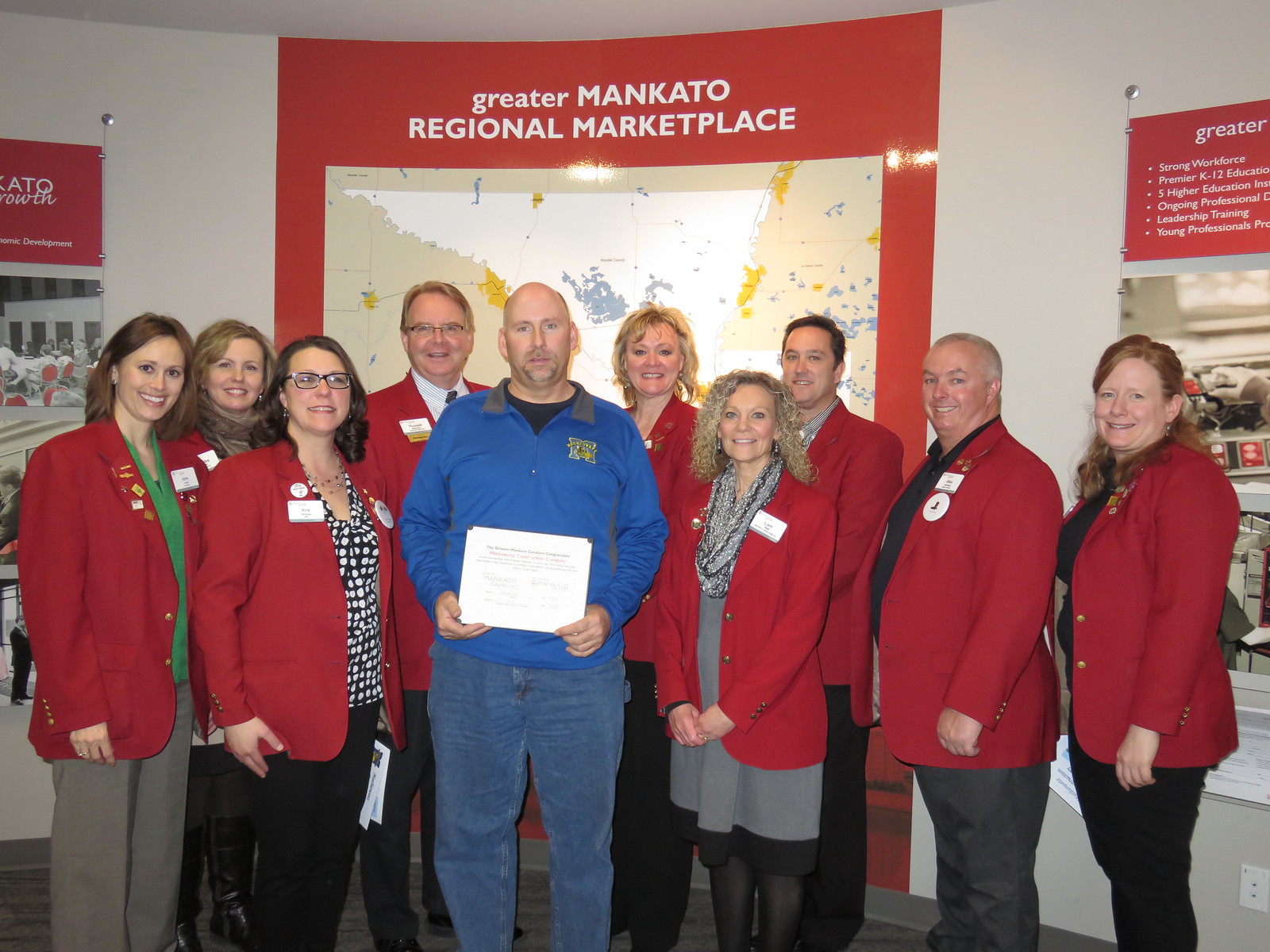In this vibrant group photo, a middle-aged man stands at the center, wearing a blue jacket over a blue dress shirt and jeans, proudly holding a certificate. He is surrounded by nine other individuals, all clad in red jackets, which appear to be their uniform. The group, consisting of both men and women, is beaming happily. Behind them, a sign with a map and three large graphics stands out, the central graphic being a map with the words "Greater Mankato Regional Marketplace" in bold red letters. Banners flank this central sign, adding to the celebratory atmosphere. Everyone in the photo is in business attire under their uniforms, adding to the professional yet cheerful vibe of the scene.